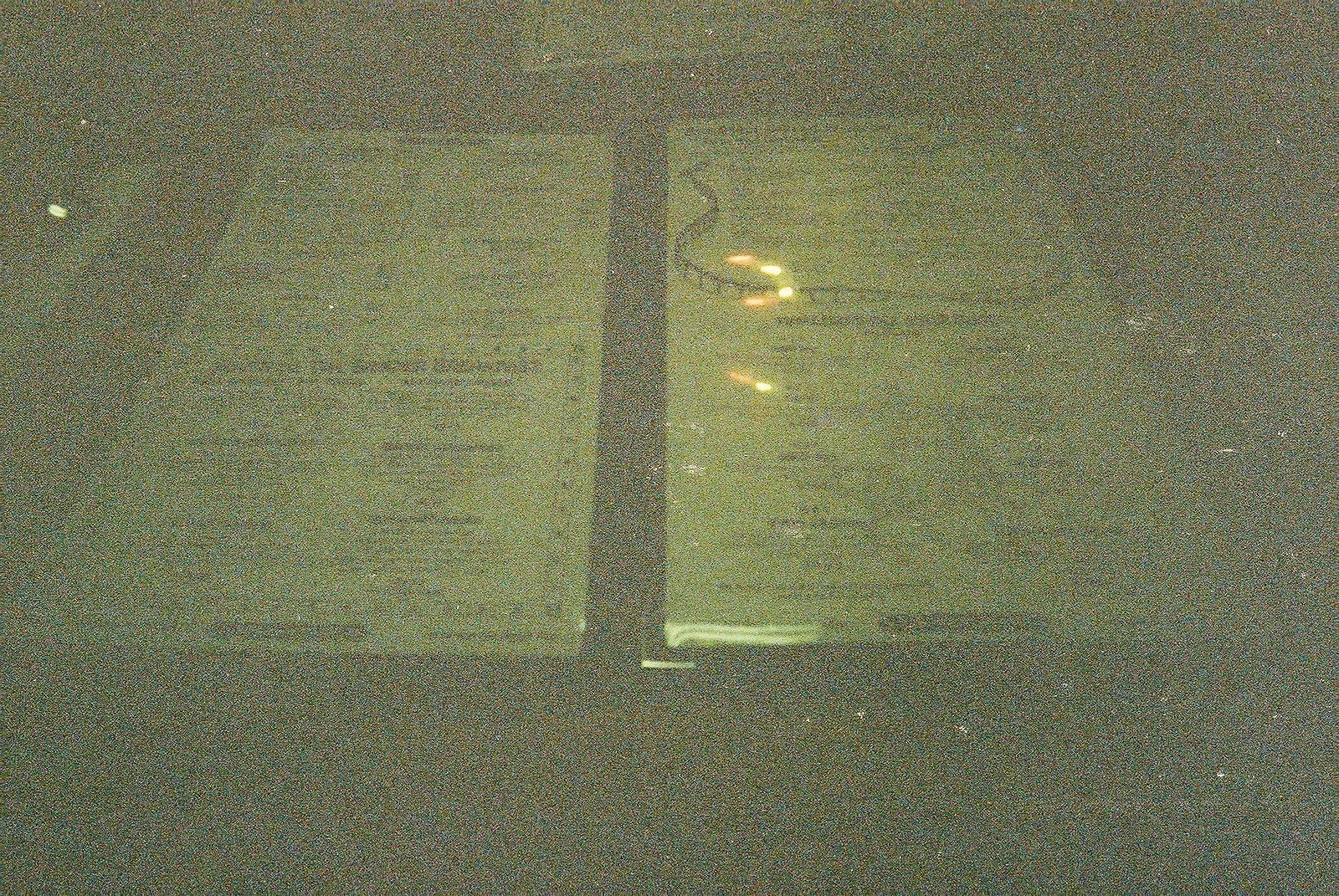A dimly-lit photograph captures a menu at a low-light restaurant. The menu, seemingly made of plastic, is difficult to discern due to the darkness of the image and the reflection of overhead lights. Despite this, it is evident that the menu is divided into several sections, possibly featuring main courses and other items. The right-hand side of the menu includes some drawings alongside the list of items. On the left-hand side, there is a drawing resembling unraveling film, which runs along the border of the menu. Five lights reflect off the plastic surface of the menu, adding to the obscurity of the image. The menu rests on what appears to be a table in the restaurant.